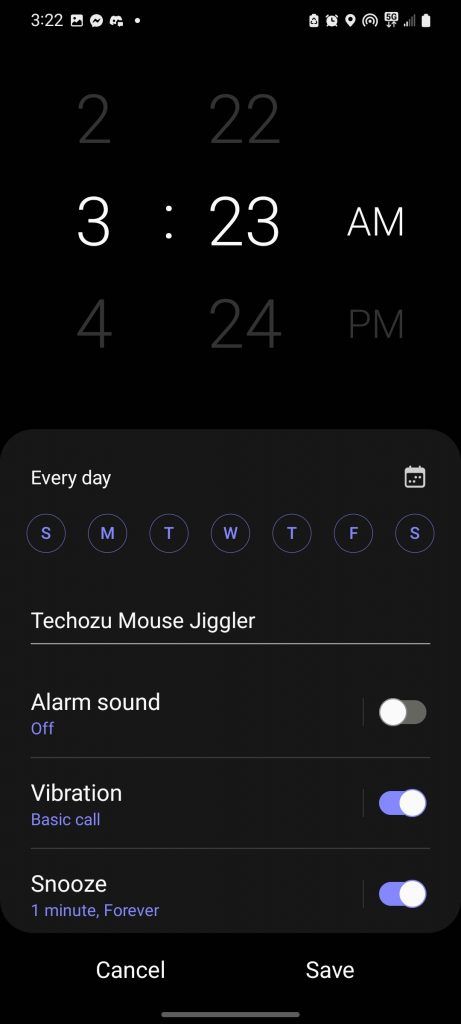The image depicts an alarm clock interface with various settings. At the top of the image, there are three displayed times: the top and bottom times are 2:22 (in grey) and 4:24 p.m. (in grey), respectively. The middle time, shown in white, is 3:23 a.m. This middle alarm is the active one.

Below the time displays is a settings panel. The alarm is set to repeat every day of the week, with each day from Sunday to Saturday written in blue circles. Below this, the alarm sound is labeled as "Tekozo Mouse Jiggler." However, the alarm sound is currently turned off, as indicated by a grey toggle switch pushed to the left. 

The next setting is for vibration, which states "Basic Call." The vibration feature is turned on, with its toggle switch pushed to the right and colored blue. The final setting involves a snooze function that is labeled "Snooze for 1 minute forever," which is also active, as shown by the blue toggle switch pushed to the right.

At the bottom of the settings panel, there are two buttons: "Cancel" and "Save," both written in white text. This detailed arrangement offers a comprehensive view of the alarm settings and configurations.